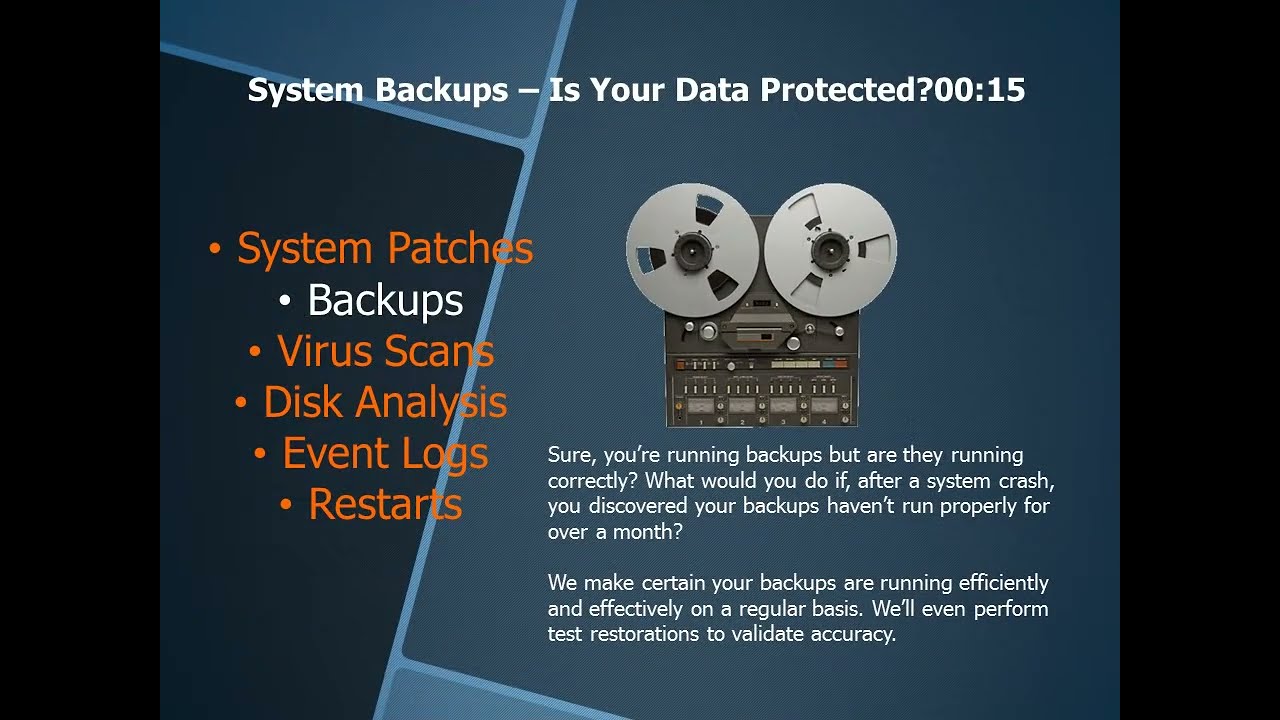**Detailed Caption:**

The image is a richly colored slide, predominantly in a gradient of navy and teal, featuring the title "System Backups: Is Your Data Protected? 00:15" in bold white text at the top. The slide has a structured layout with a clear dichotomy between the content on the left and the visual elements on the right. On the left, there is a list of bullet points highlighting key aspects of system maintenance, each bullet preceded by an orange dot except for "Backups," which is in white: 

1. System Patches (orange)
2. Backups (white)
3. Virus Scans (orange)
4. Disk Analysis (orange)
5. Event Logs (orange)
6. Restarts (orange)

To the right of this list, there is an illustration resembling a vintage reel-to-reel tape recorder, depicted with two large circular reels mounted on a metal board and several knobs and controls beneath it. This illustration evokes a sense of meticulous data handling and vintage technology.

Below the illustration, the slide includes two explanatory paragraphs in white text. The first paragraph brings attention to the importance of verifying backup integrity: "Sure, you're running backups, but are they running correctly? What would you do if after a system crash, you discover your backup hasn't run properly for over one month?" The second paragraph reassures the audience: "We make certain your backups are running efficiently and effectively on a regular basis. We even perform test restorations to validate accuracy."

The overall background features subtle geometric shapes, adding a modern and sleek aesthetic. Thick black borders frame the left and right edges of the slide, giving it a polished, professional appearance.